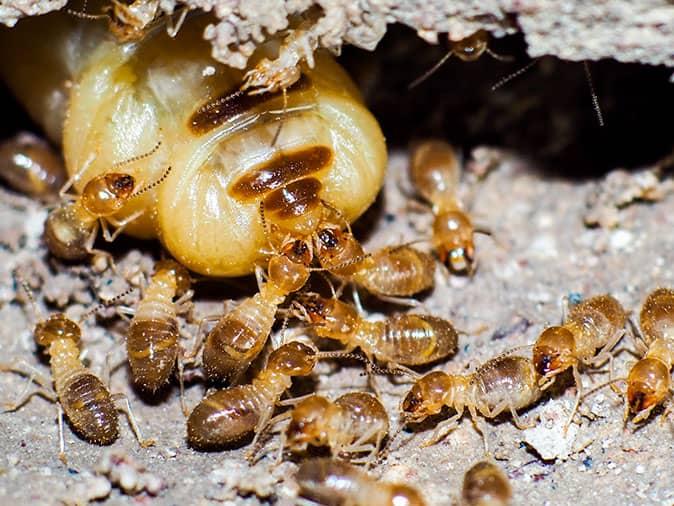This is a highly detailed macro photograph of a number of small, tan and brown segmented insects, likely termites, situated on a sandy and rocky ground surface. The scene includes an evident overhanging section of earth along the top of the image, with termites hanging upside down, walking on the ceiling of this overcropping. Approximately 15 termites are sharply in focus, with a few more visible in the blurred background, actively moving around. Central to the scene is a much larger, light ivory pupa or larva, partially visible as it emerges between the two layers of earth. Several termites appear to be grasping at the head of this pupa or larva with their pinchers, though it remains unclear if they are consuming it. The ground surface suggests a well-lit outdoor setting, contrasting with the shadowy overhang, emphasizing the vividness and activity of this natural termite colony.